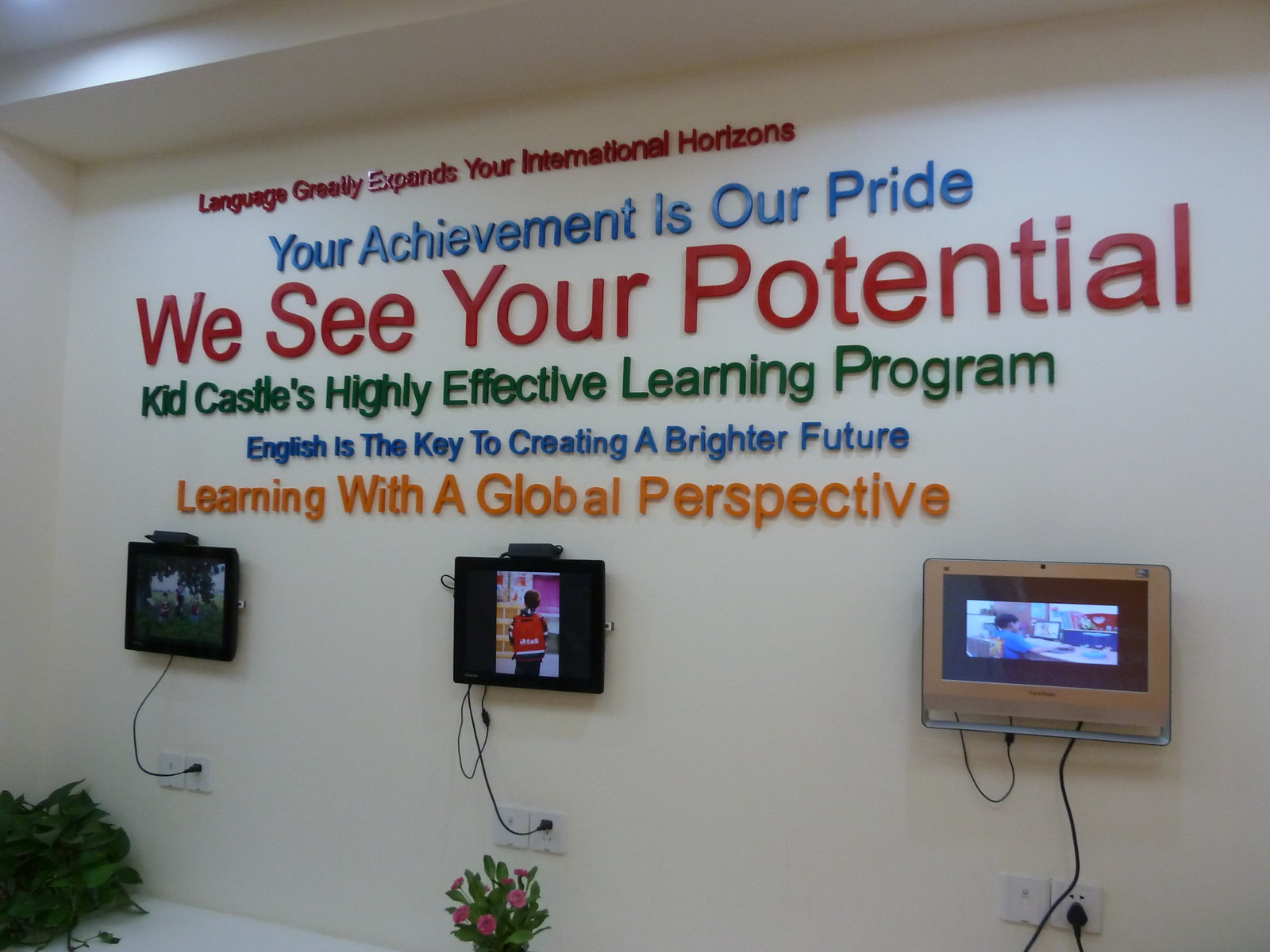This photograph captures the interior of a well-lit room with a white, beige-ish wall adorned with colorful, raised text. The text at the top of the wall emphasizes the importance of language learning and reads: "Language greatly expands your international horizons." Below this, in different colors, are the phrases: "Your achievement is our pride," "We see your potential," "Kidd Castle's highly effective learning program," "English is the key to creating a brighter future," and "Learning with a global perspective." Mounted on this wall are three monitors, each plugged into an outlet beneath them, displaying varied, indistinct images likely due to the angle and resolution. The monitors vary in color, with two black and one silver on the far right. Additionally, there are two green plants visible at the bottom left corner of the image, adding a touch of nature to the otherwise technology-focused setting.